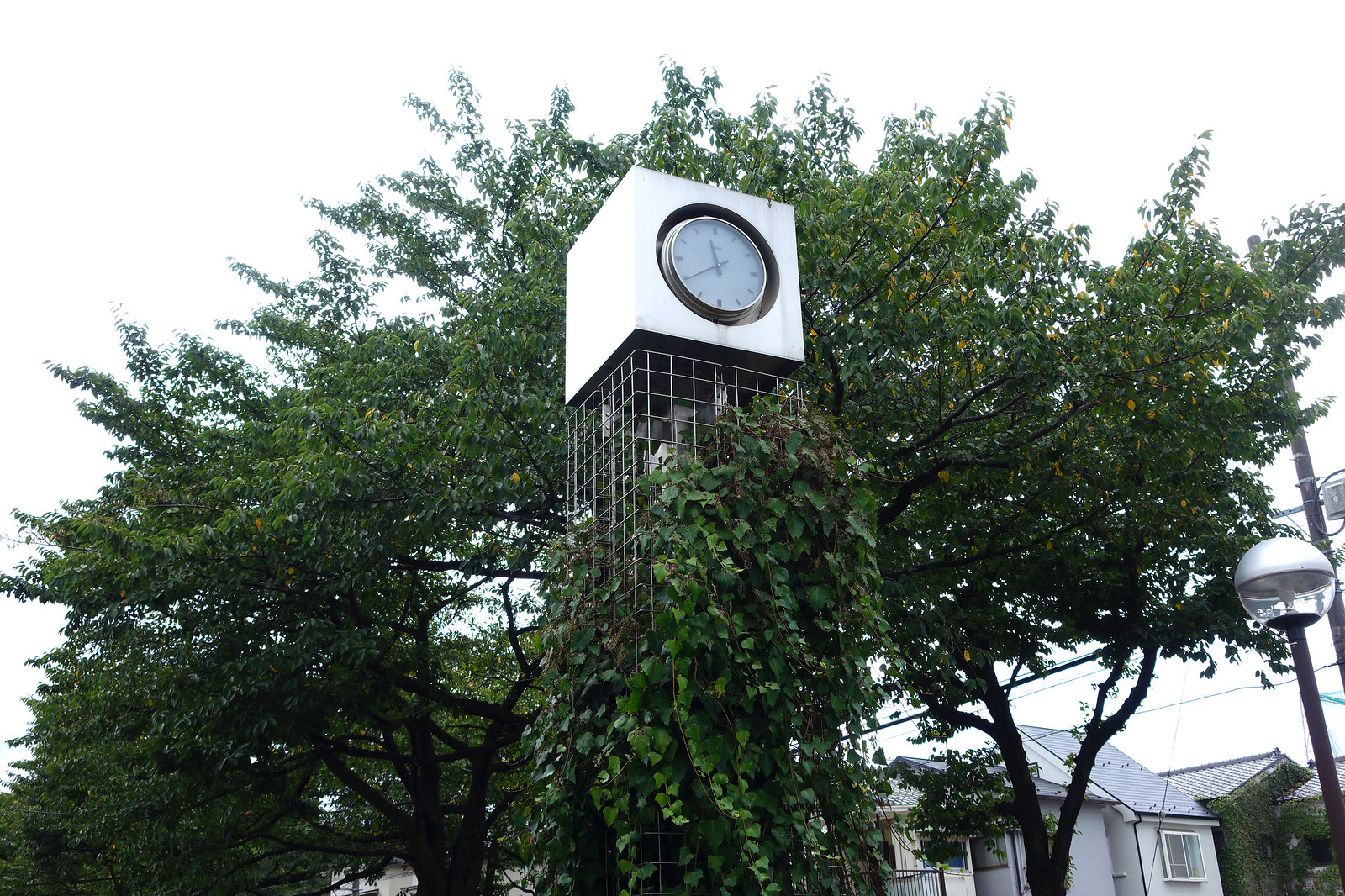The image features a whimsical clock set within a unique, cage-like structure that extends upwards, enveloped in lush greenery. Atop this ornate cage sits a pristine white cube housing a minimalist clock. The clock itself boasts a sleek silver rim and a white face marked only by simple dashes in place of numerals, reading the time as 11:40. Surrounding the structure is abundant foliage, contributing to a serene natural ambiance. The sky above is a soft white, offering a gentle contrast to the vibrant greenery. In the background, a scattering of white houses, visible in the bottom right corner, and a network of power lines add subtle hints of human habitation. A solitary light post is also discernible on the right-hand side, completing the idyllic yet slightly surreal scene.